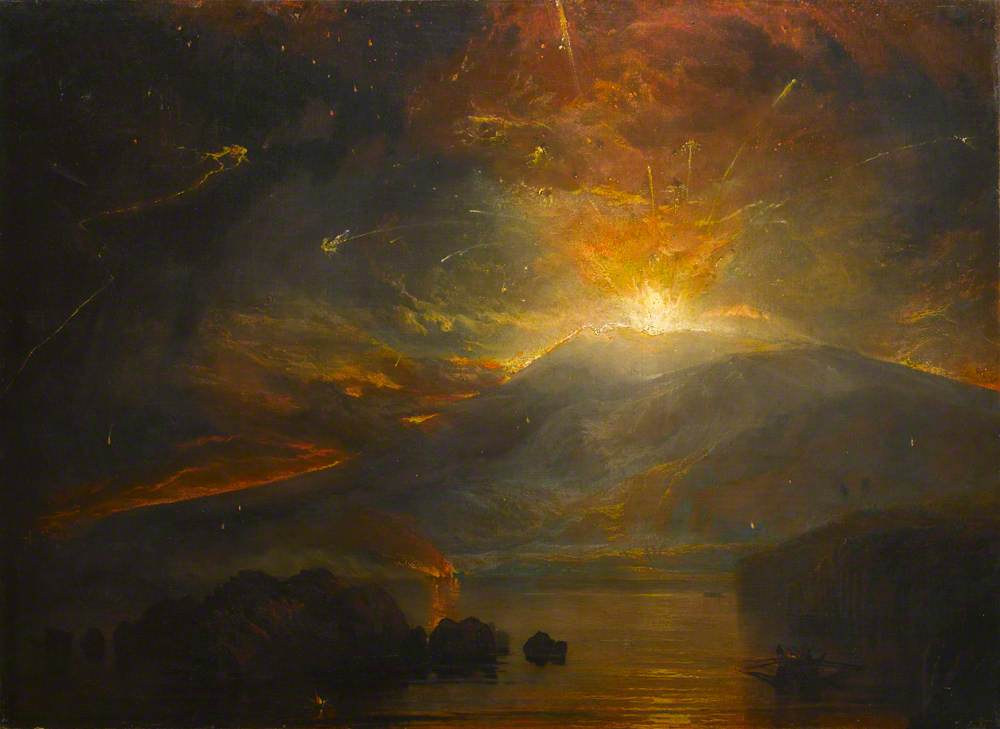The painting titled "The Eruption of the Soufriere Mountains in the Island of St. Vincent," created in 1812 by Joseph Mallord William Turner, is a vivid landscape capturing the dramatic eruption of a volcano at night. The main focus is the volcano, positioned towards the center right, erupting with a bright, fiery burst into a cloud of reddish smoke. The sky above is dark, ranging from deep blue to black, punctuated by dark clouds and illuminated by the golden glow around the volcano's base. Fiery streaks of debris shoot from the volcano's summit, adding to the chaos of the scene. To the left, lava flows down the mountain's side. 

In the foreground, a body of water, possibly a lake or the ocean, reflects the intense orange flames, creating a striking contrast with the dark tones of the sky and landscape. Within the water, there are indistinct, dark shapes that could be rocks, small islands, or even a boat, adding a sense of mystery. The painting, in an Impressionist style reminiscent of Thomas Cole, captures the raw power and beauty of the volcanic eruption, emphasizing the night scene filled with clouds of ash, smoke, and overwhelming volcanic activity.